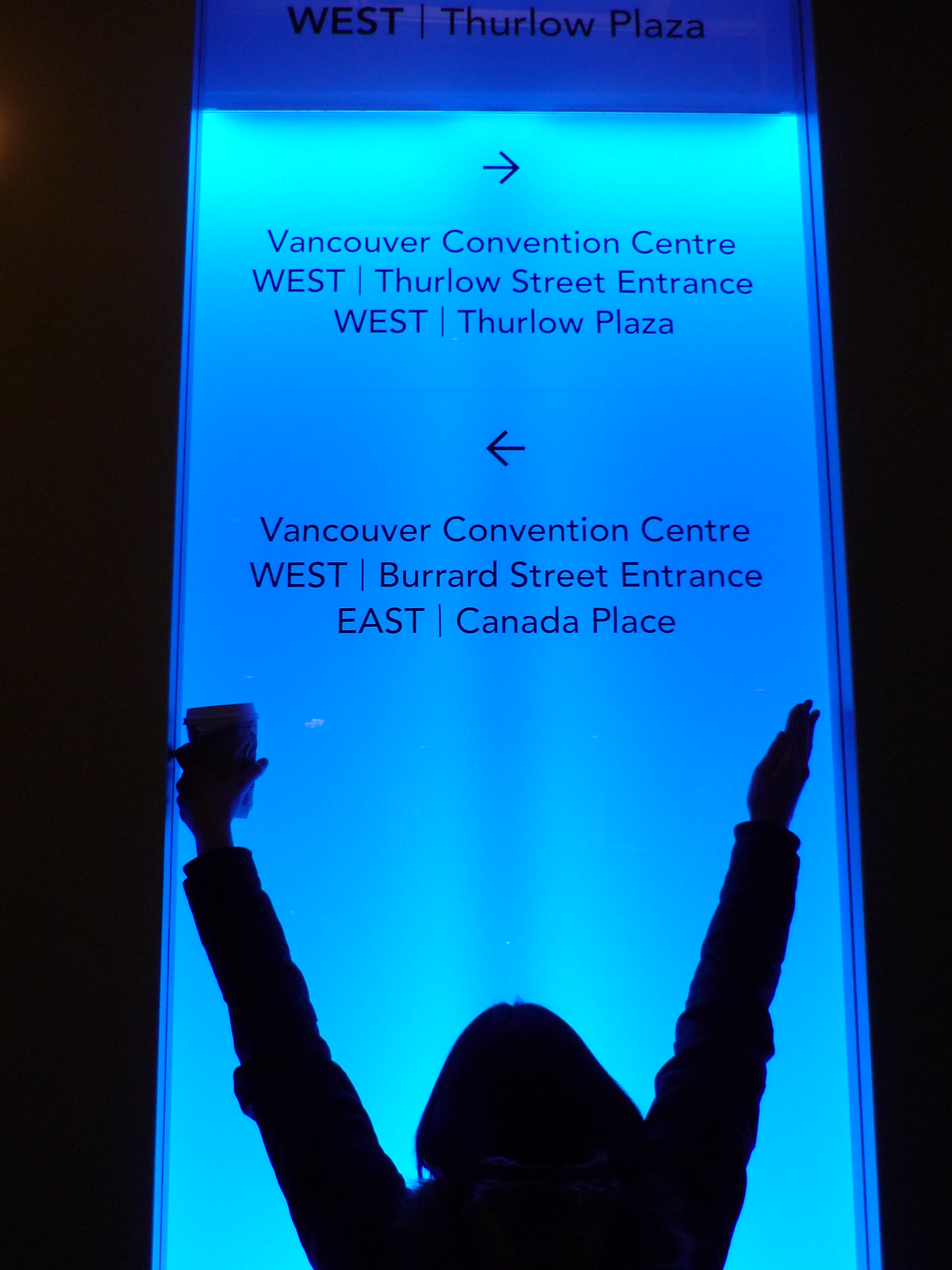In this image, a woman stands in the shadows with her arms raised, flat-palmed, towards a brightly lit directional sign. She holds a plastic coffee cup in her left hand and wears a jacket. The sign, illuminated in varying shades of blue, starts with a darker blue section at the top that reads "West" and "Thurlow Plaza" in black letters. Below, an arrow points right, directing to "Vancouver Convention Centre, West Thurlow Street Entrance, West Thurlow Plaza." Another arrow points left, indicating "Vancouver Convention Centre, Burrard Street Entrance, East Canada Place." The woman's shorter-length hair and clothing colors are obscured by the backlighting. The overall bright sign contrasts sharply with the silhouetted figure, framing the scene at West Thurlow Plaza.